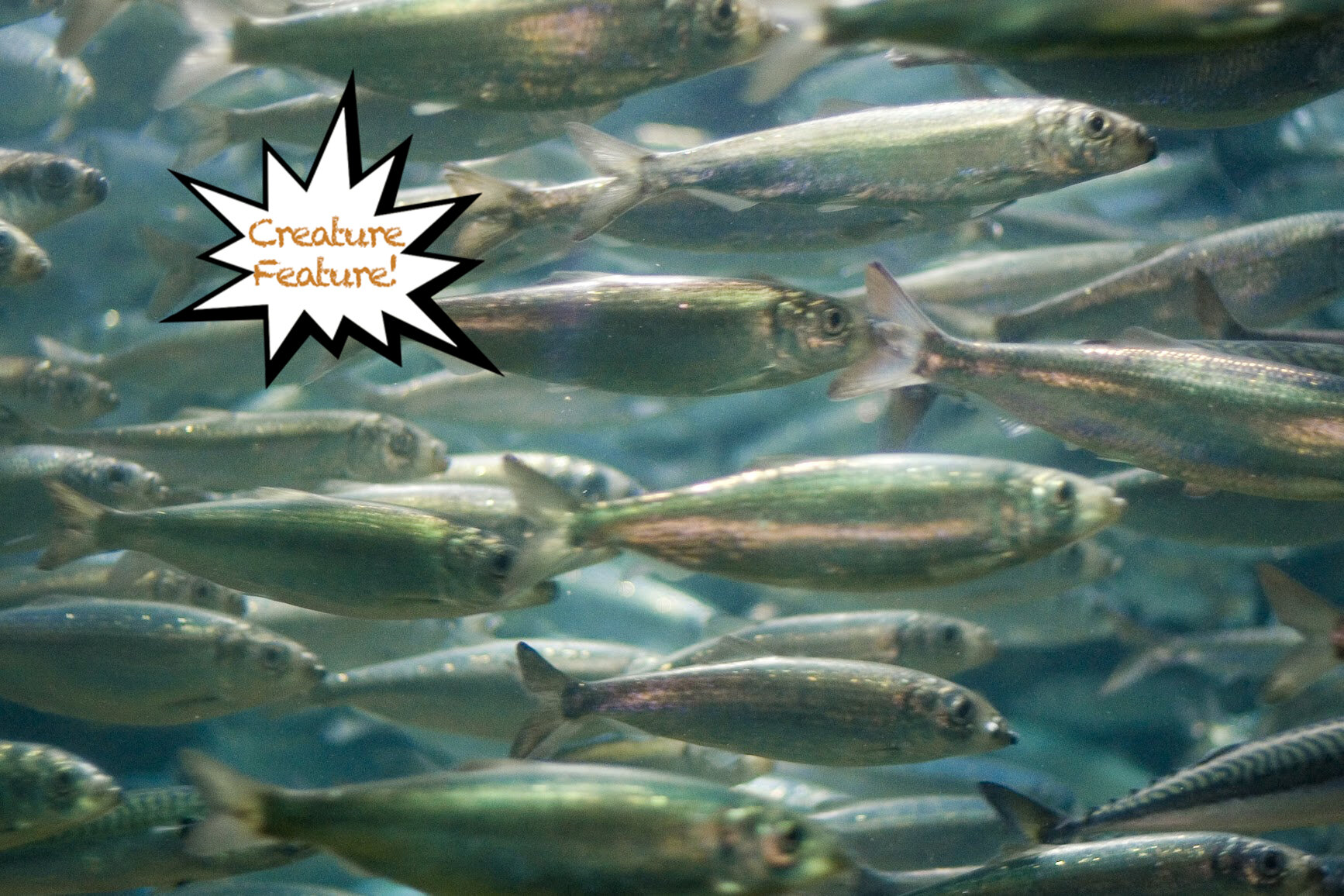The image captures a densely packed school of around 20 to possibly 50 small, macro fish in a clear aquamarine setting, similar to a pond or an aquarium. These oblong fish, each measuring about three to four inches, possess a sleek, metallic greenish body with gold and silver shimmery gills, complemented by distinctive yellow and black eyes. They are all swimming cohesively to the right, filling the entire composition. Above this aquatic scene, in the top left corner, there's a block of text within a stylized white starburst that reads "Creature Feature." The major colors in the image are varying shades of blue, white, black, brown, and green, with a noticeable yellow light filtering from the top center, suggesting natural sunlight piercing the water.